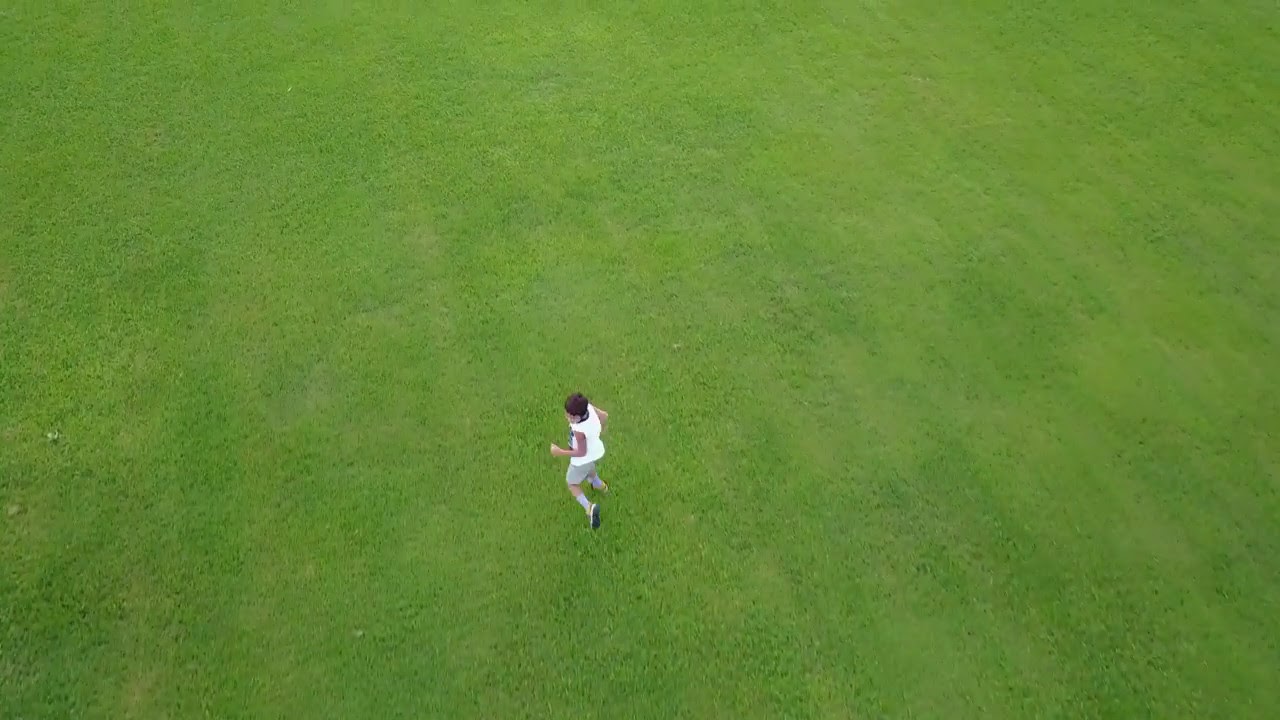The image is a detailed aerial photograph taken from about a hundred feet above, capturing a large, newly mowed grassy field with visible mowing lines. The grass covers the entire frame, showcasing variations in its green hues, with some patches appearing slightly less vibrant but healthy. In the center of the image, a boy, likely around nine years old, is caught mid-jump or in a running pose, creating a sense of dynamic movement. He is dressed in a white cotton tank top, gray shorts that fall just above his knees, gray mid-calf socks, and tennis shoes with black soles that appear brown. His short brown hair grazes his eyebrows and ears, and he has a light complexion. The boy's left foot is lifted, and his left arm is bent at the elbow in a typical running posture, adding to the realism and vividness of this drone-captured scene.